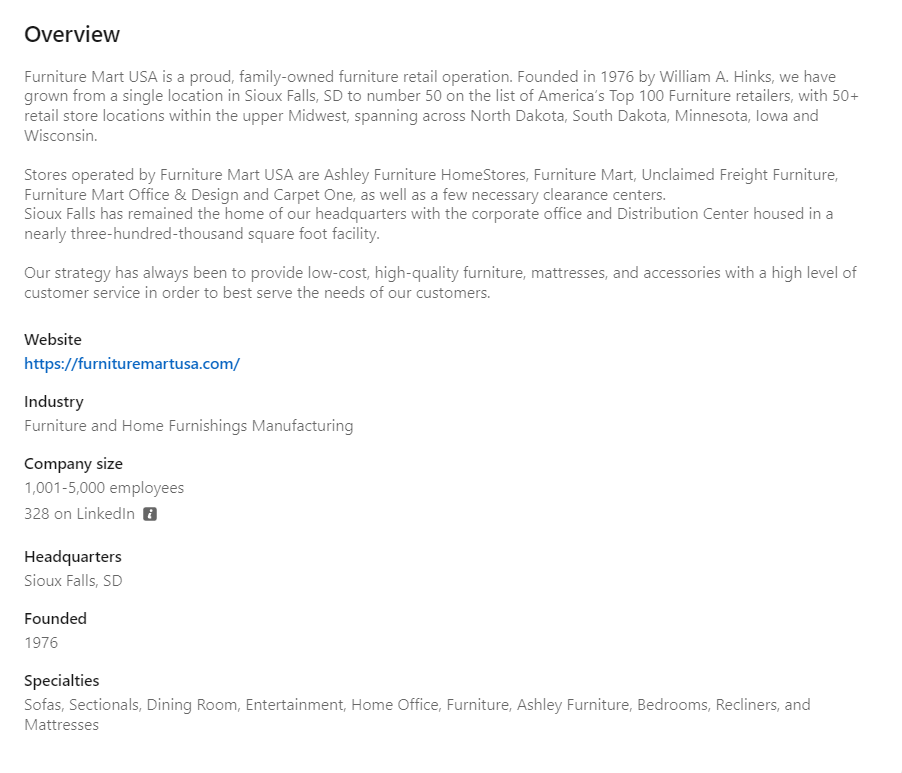**Detailed Caption for a Website Screenshot:**

*Screenshot of Furniture Mart USA's website showcasing the "Overview" section. The website highlights the company's evolution and achievements:*

*Furniture Mart USA, a family-owned furniture retail operation founded in 1976 by William A. Hinks, proudly traces its roots to a single location in Sioux Falls, South Dakota. Over the decades, it has expanded impressively, earning the 50th spot on America's top 100 furniture retailers list. The company operates over 50 retail stores across the Upper Midwest, with presence in North Dakota, South Dakota, Minnesota, Iowa, and Wisconsin.*

*The stores under Furniture Mart USA's umbrella include well-known names such as Ashley Furniture Home Stores, Furniture Mart, Unclaimed Freight Furniture, Furniture Mart Office and Design, and Carpet One, along with several essential clearance centers. The company's headquarters have remained in Sioux Falls, where both the Corporate Office and a nearly 300,000 square foot Distribution Center are located.*

*Maintaining a strategy focused on providing low-cost, high-quality furniture, mattresses, and accessories, the company emphasizes exceptional customer service to meet customers' needs. The website link is https://furnituremartusa.com, and the company operates within the Furniture and Home Furnishings Manufacturing industry. Employing between 1,001 to 5,000 staff, Furniture Mart USA also has a significant presence on LinkedIn with 328 employees.*

*Established in 1976, the company specializes in a diverse range of furniture including sofas, sectionals, dining room sets, entertainment units, home office furniture, bedrooms, recliners, and mattresses.*